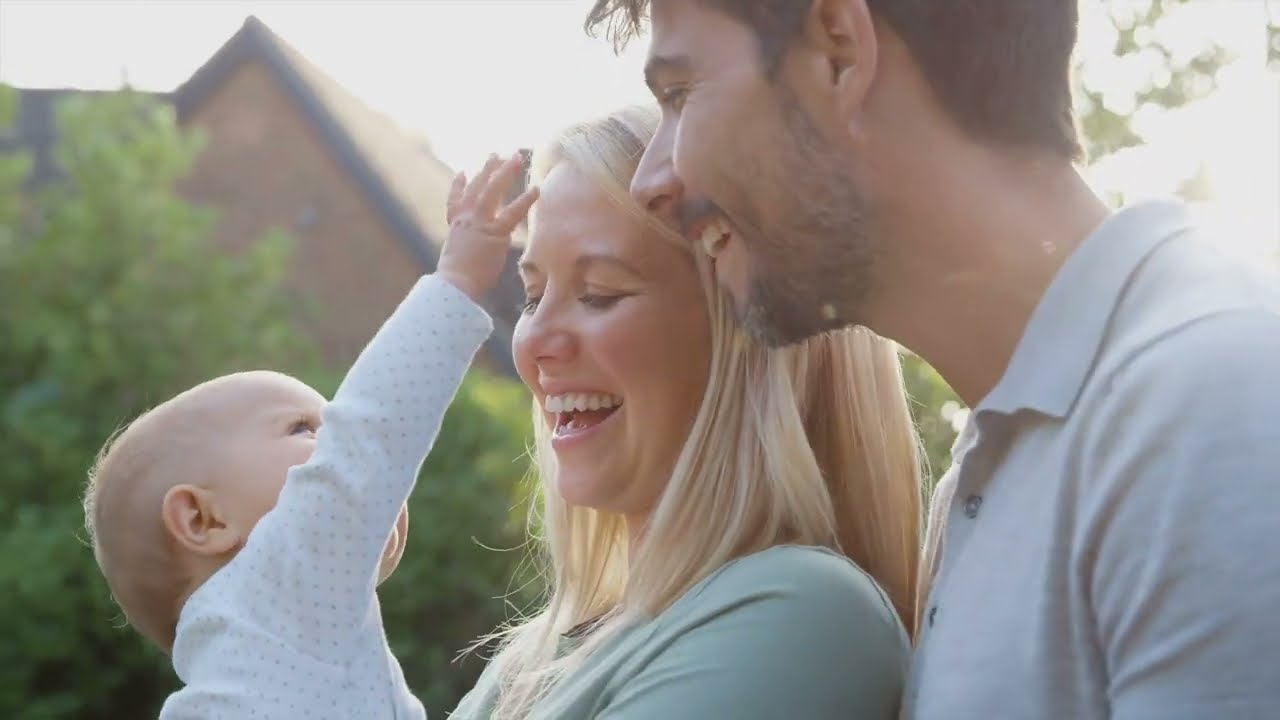In this vibrant outdoor family photo, a joyful white woman with blonde hair, dressed in a mint green shirt, stands at the center holding an infant with sparse, light hair. Both mother and baby are the focal points, with the mother beaming down at her child and the baby, clad in a white long-sleeve top with light blue dots, reaching out towards the father. The father, a white man with dark hair, a thin beard, and mustache, is positioned just behind the mother on her right side. He is wearing a gray button-up shirt and is smiling warmly at the baby. The scene is set against a blurred background featuring green foliage, predominantly on the left, and part of a brown house with black roof trim peeking through the greenery. It's a sunny day, enhancing the warmth and happiness radiating from the family.